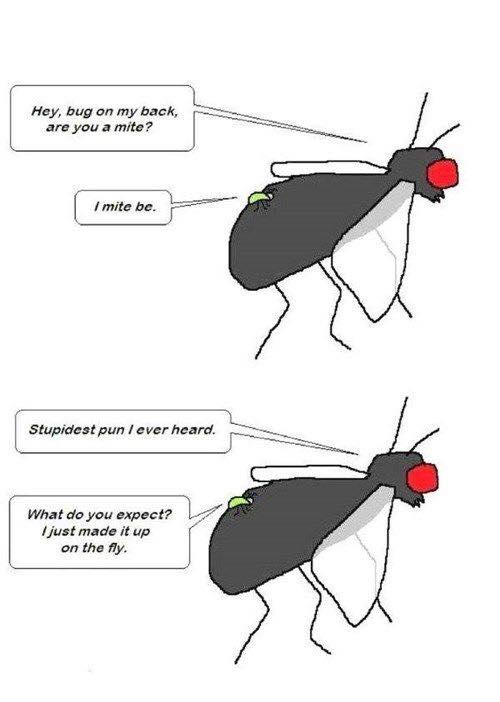The image resembles a meme or a short comic strip typical of the internet, displayed on a white background. It features two illustrations of black flies with large red eyes, transparent white wings, and visible antennas and legs. On the back of the top fly, there's a tiny light green bug. The scene is accompanied by dialogue in white text boxes with black lettering. 

In the first part, the larger fly on the top right says, "Hey bug on my back, are you a mite?" The smaller green bug on its back humorously replies, "I might be." Below this, the same black fly continues the exchange with, "Stupidest pun I ever heard," to which the tiny green bug responds, "What do you expect? I just made it up on the fly."